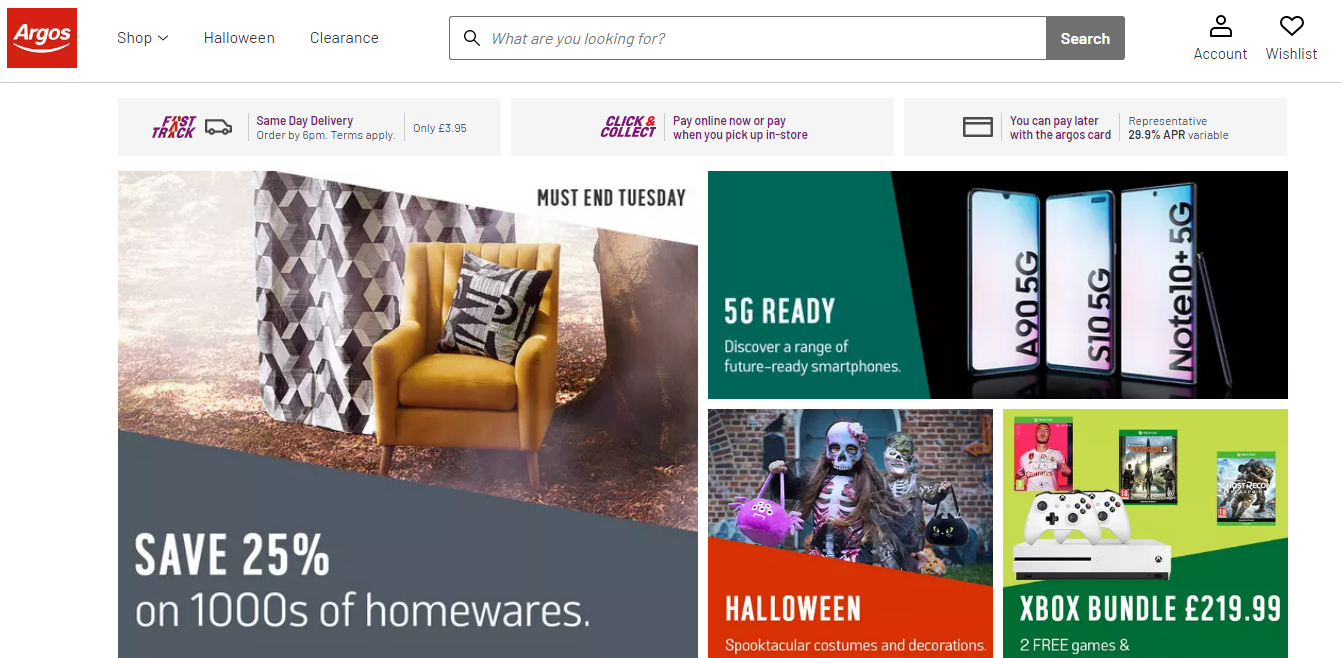The image is a screenshot of the homepage of the retail site Argos. The background color is predominantly white. In the upper left-hand corner, the Argos logo is prominently displayed, written in white text inside a red box with a small white curved line underneath it.

The top navigational bar features three main options: "Shop," "Halloween," and "Clearance," all written in a gray font. Positioned centrally within this bar is a search box. To the right are icons for "Account" and "Wishlist."

The main body of the homepage is dominated by large, attention-grabbing photos. On the left side, there is an image of a gold-colored side chair next to a curtain featuring shades of gray and black in a diamond pattern. Below this image is a white caption that reads, "Save 25% on thousands of homewares."

Towards the upper right-hand side, another photo displays three smartphones with the caption "5G Ready," followed by "Discover a range of future-ready smartphones."

Further down, there is a photo related to Halloween, showcasing children dressed up in various costumes. On the lower right-hand corner of the homepage is an image of an Xbox Bundle priced at £299.